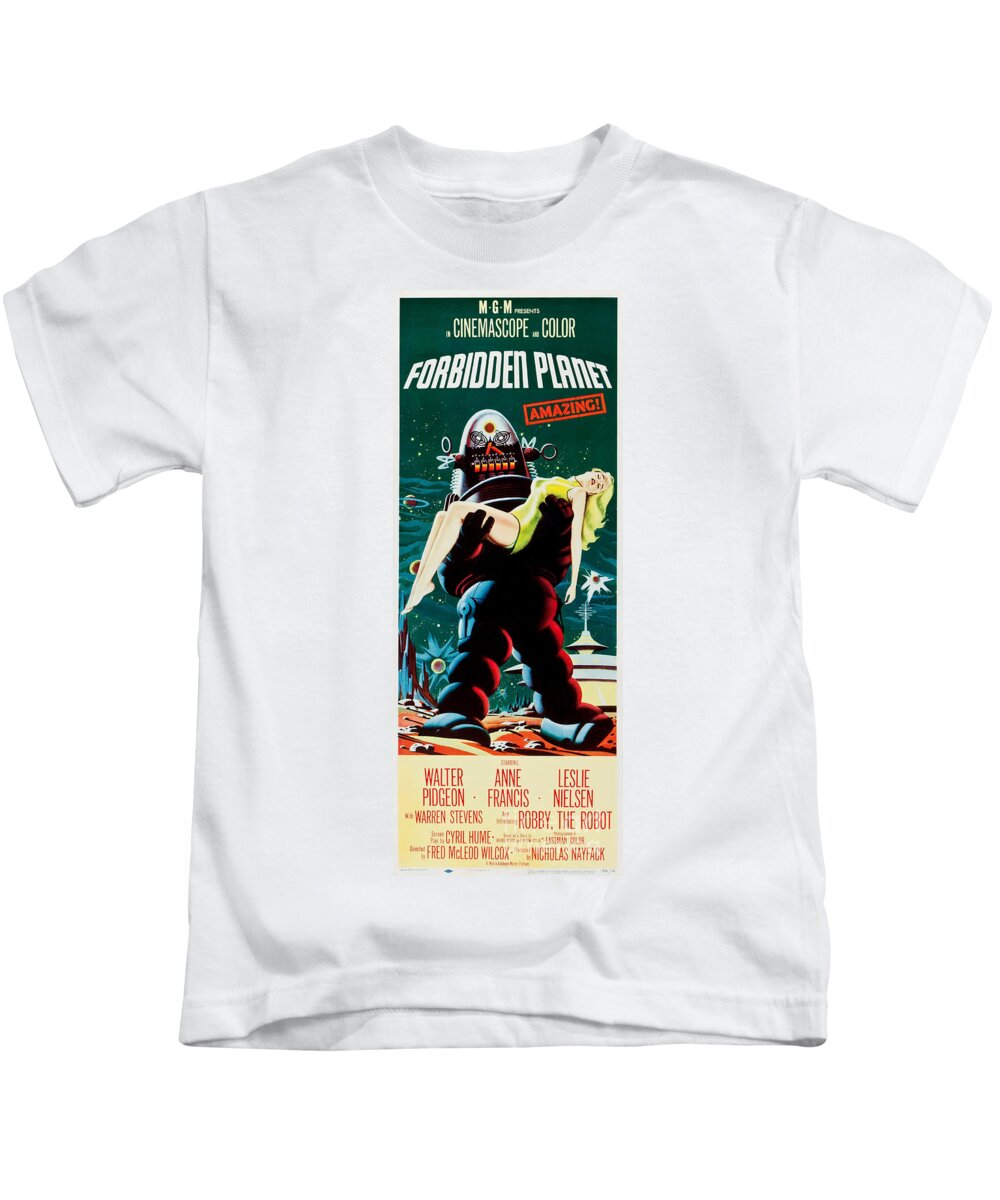The product image showcases a white T-shirt set against a solid white background. The shirt features a vintage 1950s movie poster for the science fiction classic, *Forbidden Planet*. At the top of the poster, prominently printed in large white font, is the title "Forbidden Planet," with "Cinemascope Color" noted above it. The central artwork on the T-shirt depicts the iconic character Robbie the Robot, wearing a helmet and carrying a blonde woman in distress, who is dressed in a green outfit that might be a dress or bathing suit. This scene takes place on an extraterrestrial planet, indicated by the background. Below the main artwork, in red font against a yellow background, are the names of the movie's stars: Walter Pidgeon, Anne Francis, and Leslie Nielsen, with a special mention of Warren Stevens and Robbie the Robot. While the director and screenplay writer are listed at the bottom, the font is too small to read clearly. The design is set in a narrow rectangular format that runs vertically down the center of the shirt.